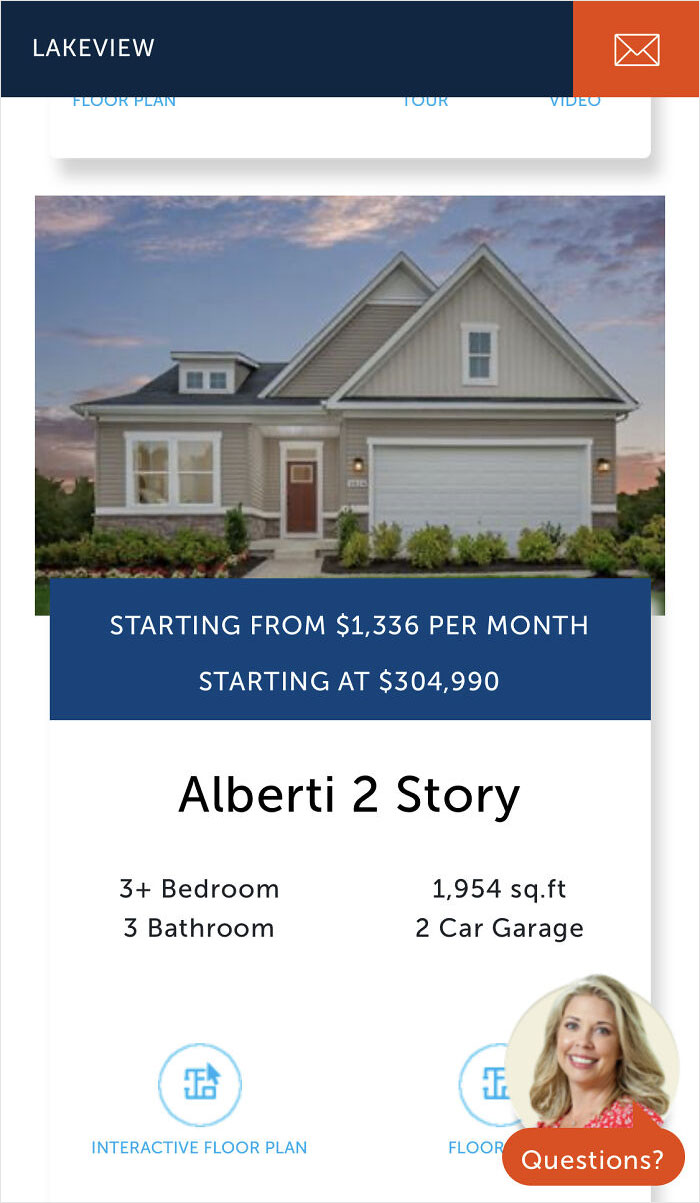Screenshot of a real estate listing for a house. Here's the detailed breakdown:

- **Top Section:**
  - At the top left, there's a black bar with the text "Lakeview" in white, situated on the left-hand side.
  - Adjacent to the black bar is an orange square featuring a white envelope icon.

- **Main Background:**
  - The background is predominantly white.
  - A faint, partially visible pop-up, written in blue text, reads "Floor Plan Tour in Video."

- **House Image:**
  - The central image showcases a very nice ranch-style, single-story house under a baby blue sky.
  - The house has tan siding and appears to have a one or two-car garage, although there are plants planted in front, suggesting the garage may not be used for parking.
  
- **Price and Details:**
  - Below the image, there is a blue rectangle with white text stating "Starting from $1,336 per month starting at $304,900." This suggests mortgage options for the property.
  - Additional information on a white background reads "Aberdeen Two-Story," even though the image depicts a single-story house. The listing specifies "Three plus bed, 1,954 square feet, three bedroom, three bath."

- **Agent Information:**
  - An image of a generic person with fake blonde hair smiling.
  - Right below the image of the agent, there is a pop-up box labeled "Questions."

This well-organized screenshot gives a detailed overview of a house listing, including the property details, financing options, and a contact feature for inquiries.